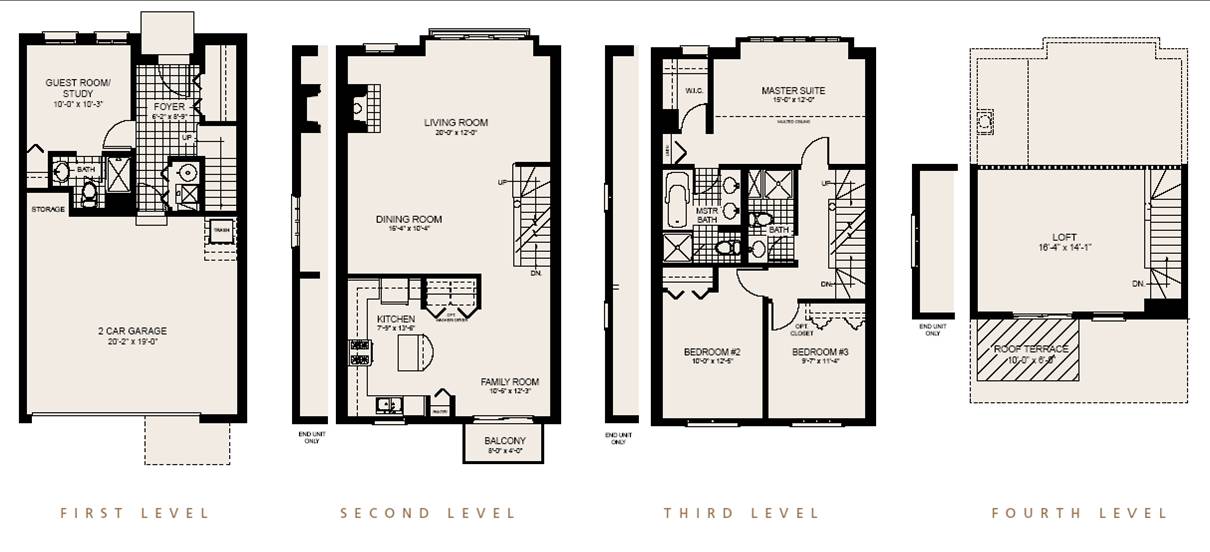The image features a detailed side-by-side layout of the four-floor plans of a house, each representing a different level and labeled accordingly as "First Level," "Second Level," "Third Level," and "Fourth Level."

**First Level (Leftmost Plan):**
- **Top Left:** Guest Room/Study
- **Top Right:** Foyer
- **Bottom:** Two-Car Garage with specified dimensions.

**Second Level (Second from the Left):**
- **Top:** Living Room
- **Middle Below Living Room:** Dining Room
- **Middle Bottom:** Kitchen
- **Right of Kitchen:** Family Room
- **Bottom:** Balcony with dimensions in tiny, nearly unreadable print.

**Third Level (Second from the Right):**
- **Top:** Master Suite
- **Middle:** Two distinct bathroom areas
- **Bottom Left:** Bedroom Number Two
- **Bottom Right:** Bedroom Number Three
- Dimensions are mentioned but in very small print.

**Fourth Level (Rightmost Plan):**
- **Middle:** Large Loft Area
- **Bottom:** Roof Terrace
- Adjacent to the Roof Terrace appears to be another space, possibly a balcony, but the label is unclear.